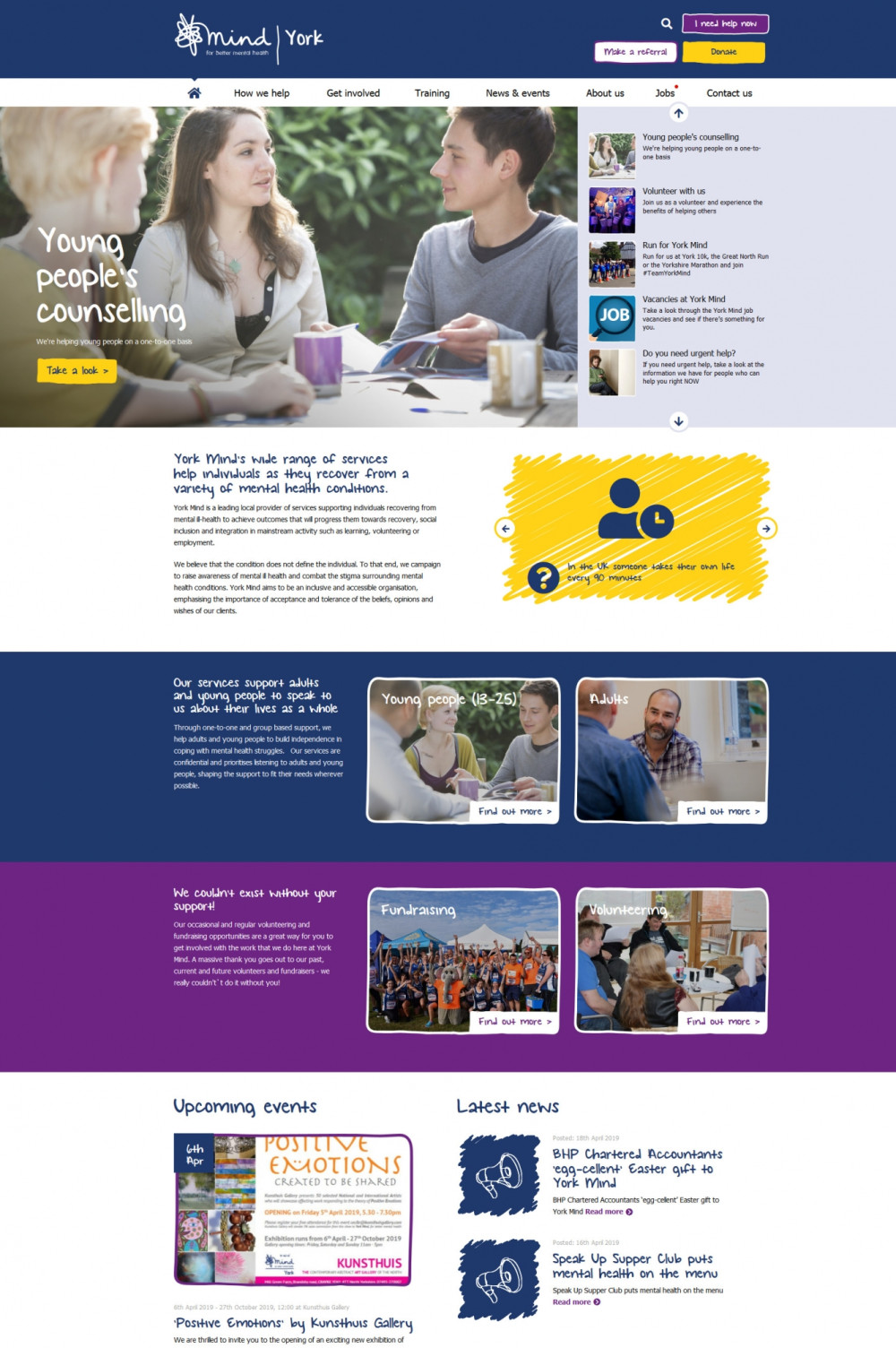The image depicts a webpage for a mental health program by the company Mind York, dedicated to improving mental health. At the top of the page, a blue banner features the company's name, "Mind York," alongside their slogan, "for better mental health." The banner also contains a white scribble logo on the left. On the right side of the banner, there are three clickable options: "I Need Help Now" (purple button with white outline), "Donate" (yellow button with blue outline), and "Make a Referral" (white button with purple outline).

Below the banner, there are navigation tabs for different sections of the website: Home, How We Help, Get Involved, Training, Meet and Events, About Us, Jobs, and Contact Us, with the Home tab currently active. The main image showcases a group of three people sitting at a table and engaging in a discussion. A yellow button overlaid on the image says, "Young People's Counseling, Take a Look."

To the right of this central image, there are various clickable articles. Farther down the page, there are several sections with text, accompanied by the website's main colors of blue, yellow, and purple, specifically dark blue and dark purple.

Towards the bottom of the webpage, there are sections for "Upcoming Events" and "Latest News." Above these, the site includes sections for different services like counseling and support groups, opportunities for fundraising and volunteering, and information tailored to adults and young people. The layout is rich with navigational links to guide users through the numerous resources available on the website.